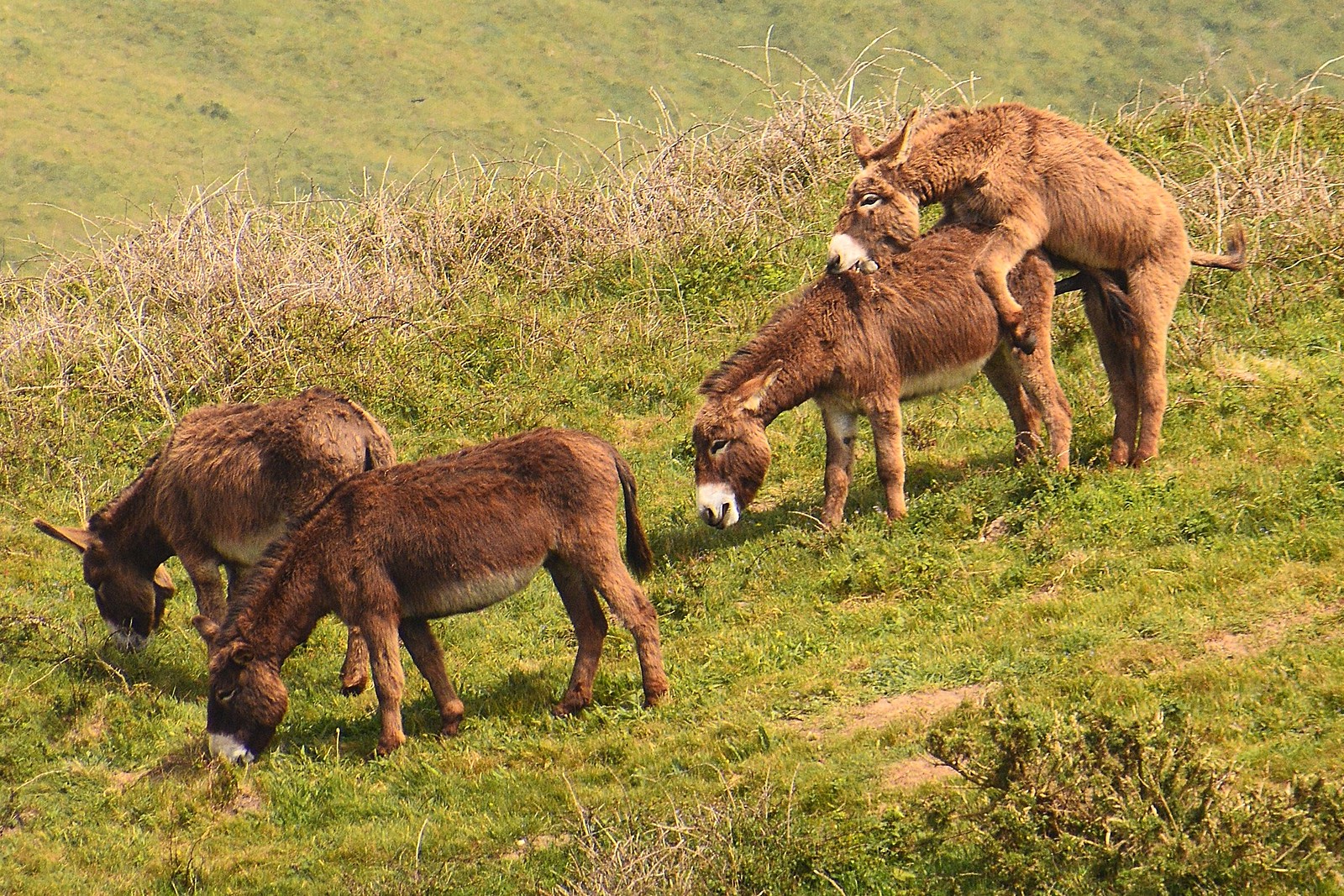In this outdoor digital photograph, the scene is dominated by a lush, green hill in the background, which sharply contrasts with the drier, straw-like vegetation in the foreground, suggesting a valley landscape. On the bottom right corner of the image, there is a small evergreen bush, adding to the greenery of the setting. More centrally and slightly to the left, two light to medium brown donkeys with white mouths and noses are grazing peacefully on the verdant grass, with their heads lowered. Behind them, there is another donkey with darker fur, similarly characterized by a white nose and mouth. This darker-toned donkey is being mounted by yet another donkey, this one with a lighter coat. The explicit nature of the interaction is accentuated by the visibly erect state of the mounting donkey. The cherubic tranquility of the green landscape and the animals' grazing is punctuated by this more dynamic and somewhat inappropriate activity.